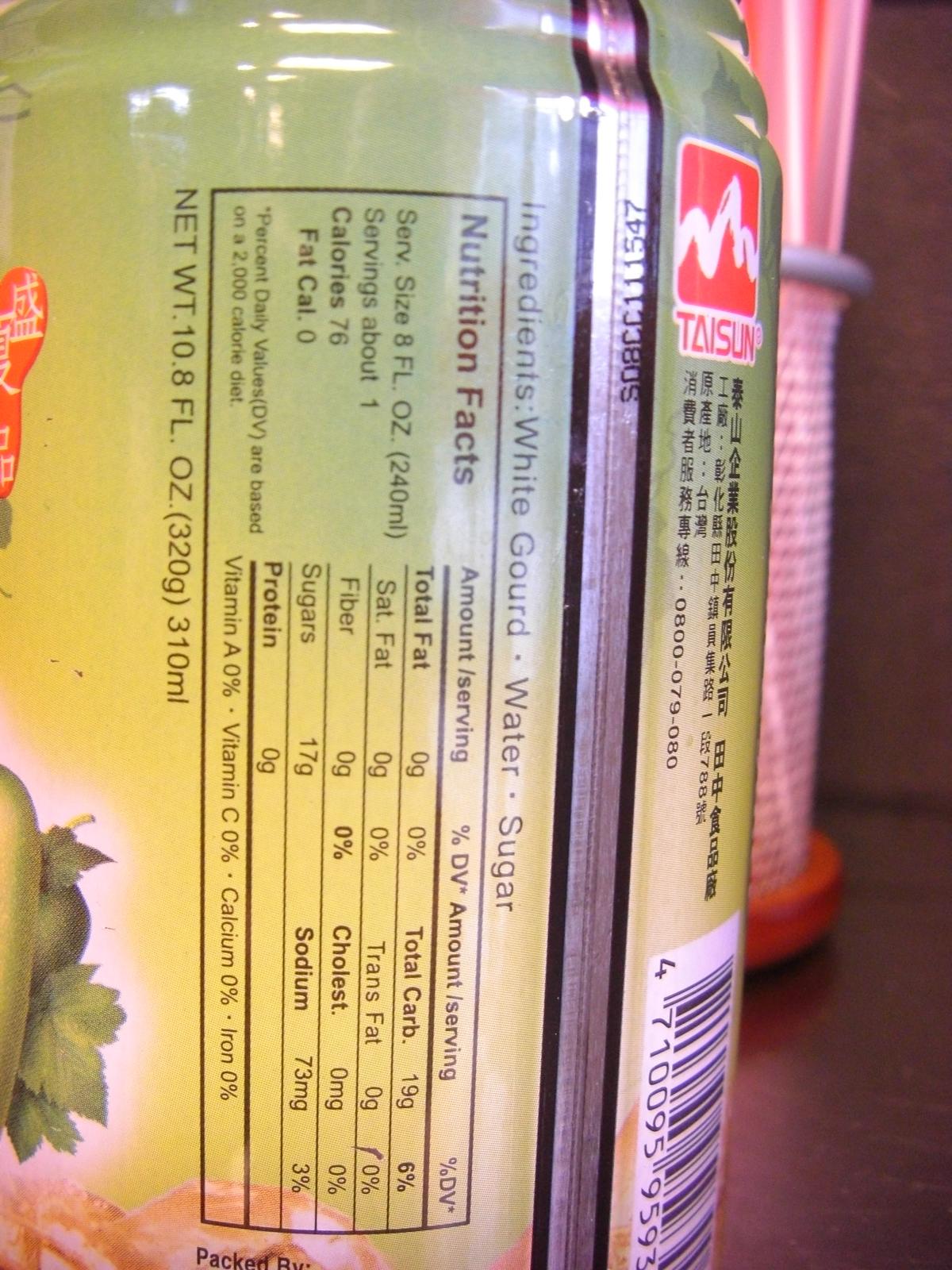This detailed image captures a side view of a tall, cylindrical bottle. The label, a striking yellowish-green, presents a comprehensive view of its nutritional information printed in a bold black font, oriented vertically. Above the nutrition information, a succinct list of ingredients reveals the contents: white gourd, water, and sugar. The nutrition facts box specifies that each serving size is 8 fluid ounces, with one serving per container. It notes that the beverage contains 76 calories with zero fat. The detailed chart below further breaks down the nutritional values, listing the serving size and percent daily value for total fat, saturated fat, fiber, sugars, and proteins. The meticulous design and clear labeling emphasize the bottle's transparency and commitment to informing consumers.